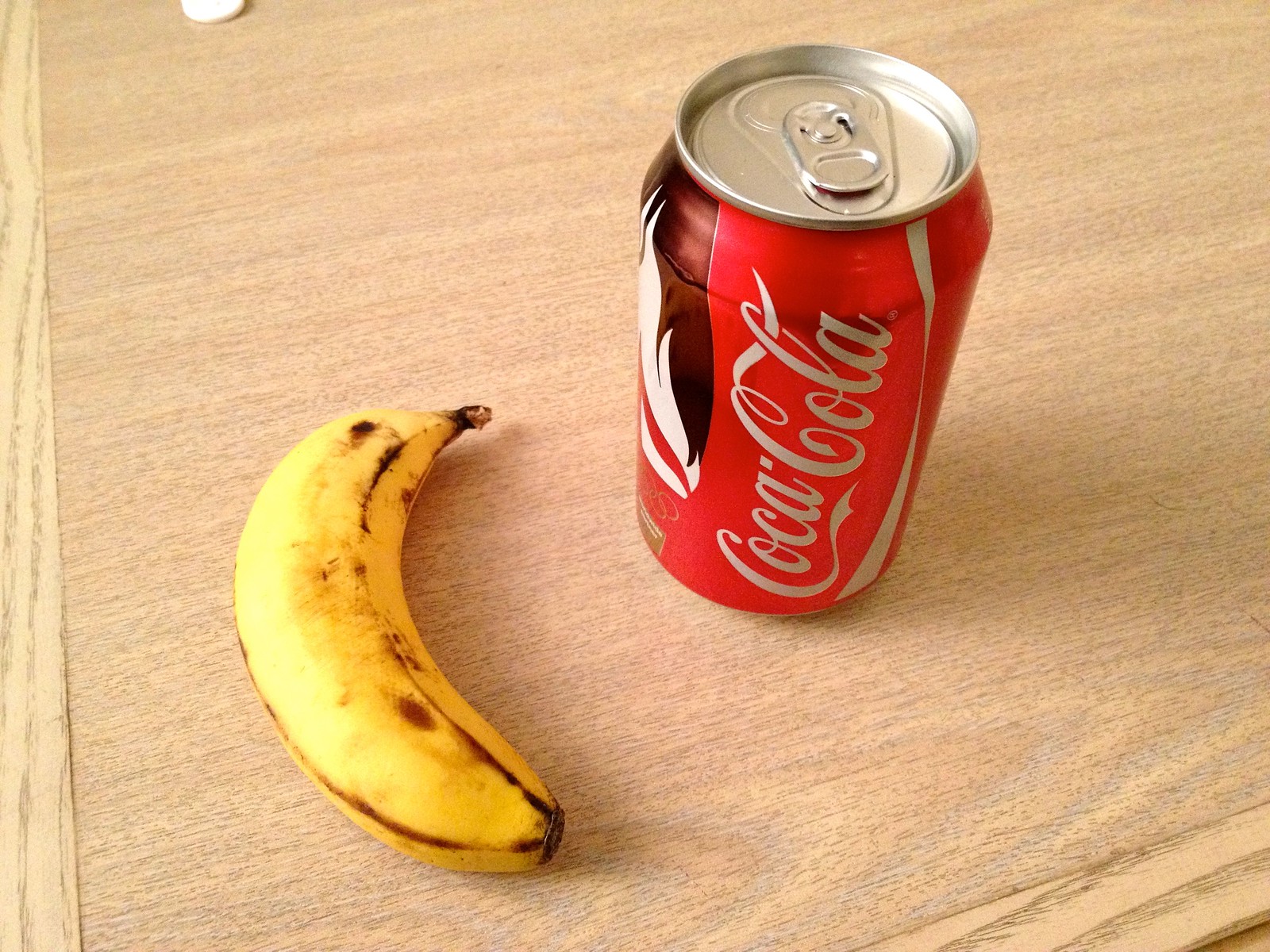On a beige wooden table, three distinct items are neatly arranged. Central to the composition, towards the edge of the table, lies a slightly overripe banana, its yellow skin freckled with brown spots, and minor browning along its curved lines. The banana curves to the left, exposing its concave side.

To the right of the banana stands a closed can of Coca-Cola. The iconic Coca-Cola logo faces forward prominently, though a small, indistinguishable brown symbol is partially visible beside it. The can also features a slight crease near the top and casts a delicate shadow beneath it, hinting at the light source streaming from the backdrop.

Above and to the upper right of the Coca-Cola can, partially off-frame, is the edge of a circular white button, resting just above the table. This subtle arrangement captures a simple yet intriguing still life of everyday objects, emphasizing their textures, colors, and the interplay of light and shadow.